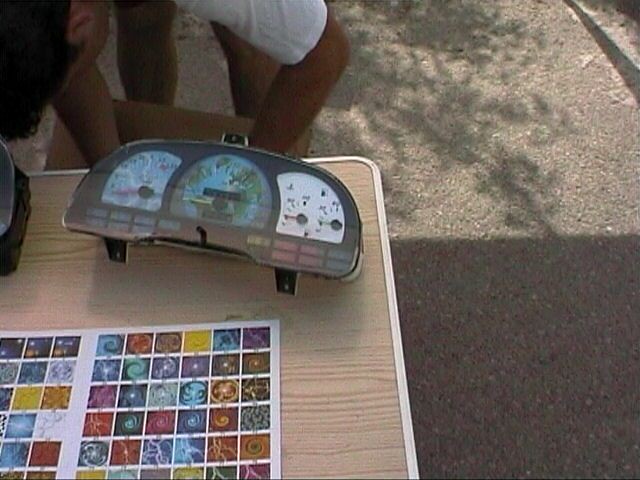The image features a boy bent over a unique wooden table, intensely examining a collection of stamps. The table's surface, made from polished wood with visible grain lines, supports an open stamp book filled with squares showcasing vibrant circular and swirly designs. Alongside the stamp book sits an antique, semi-circular measuring device with three dials, propped up by black legs. The device appears aged and used. The boy, with his head, arms, and leg visible, is deeply engrossed in his exploration of this intriguing array of patterns and tools.